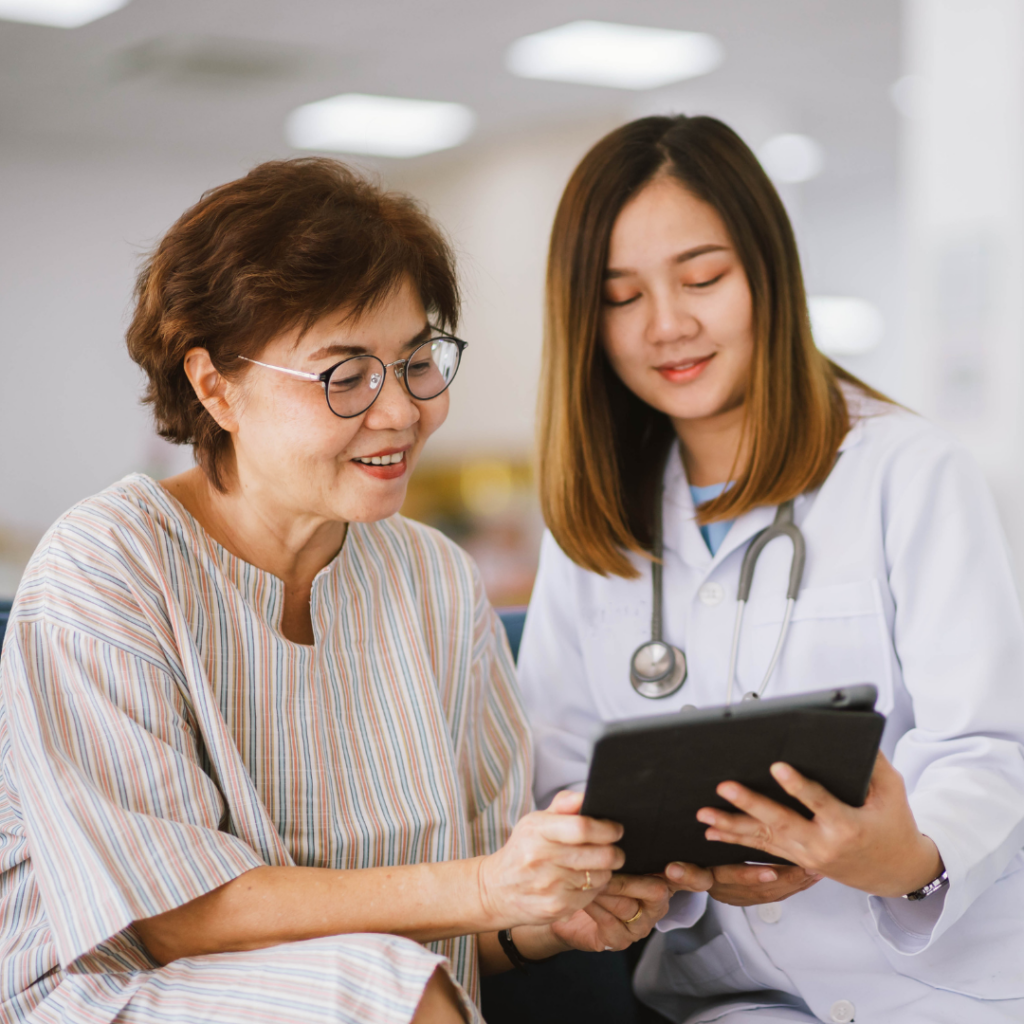In this image, we find ourselves inside a healthcare facility with bright, white lighting and white walls. The focus is on two women—one appears to be a medical professional, likely a doctor, while the other seems to be a patient. The woman on the right, assumed to be the doctor, has long brown hair cascading past her shoulders and wears a white lab coat and a stethoscope around her neck. She is looking down with a slight smile, her eyes partially closed, as she holds a tablet in her hands. She also wears a silver watch. Next to her, the patient, a middle-aged woman with shorter brown hair and black-rimmed eyeglasses, is also gazing at the tablet with a slight smile. She wears a gown with blue and pale orangish stripes. Both women appear content and are sharing the tablet, possibly reviewing medical results or discussing treatment options. The setting and their expressions suggest a moment of positive or neutral information being shared.